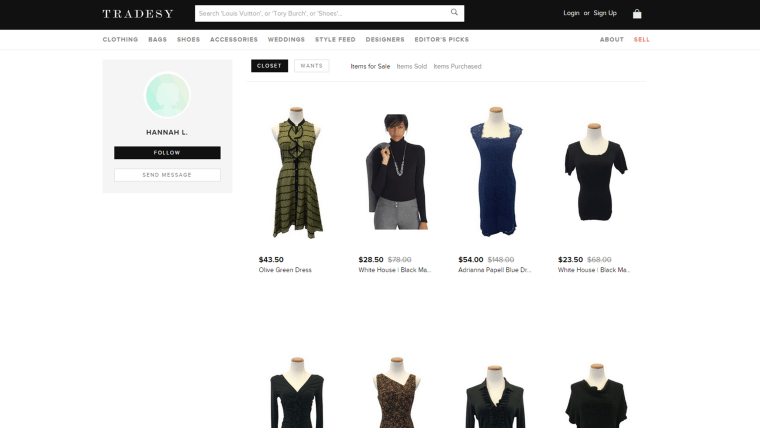Here is a cleaned-up and detailed caption for the described image:

---

The screenshot showcases the TradeZ website's homepage. At the top of the page is a black navigation bar with "TradeZ" prominently displayed in white in the upper left corner. Adjacent to the logo is a white search bar with placeholder text in light gray suggesting popular search terms such as "Louis Vuitton," "Tory Burch," or "shoes." A magnifying glass icon lies to the right of the search bar, indicating the search function.

Further to the right, in light gray text, the options to "Log In" or "Sign Up" are visible, accompanied by a shopping bag icon. Below this primary navigation bar is a secondary menu, also in gray, featuring categories such as Clothing, Bags, Shoes, Accessories, Weddings, Style Feed, Designers, and Editor's Picks, with the "Sell" option standing out in red.

To the far right of this menu is an "About" link and the "Sell" link again highlighted. The user's profile appears on the left, displaying the username "Hannah L." with a turquoise circular anonymous profile picture. Beneath the profile picture are two buttons: a black button with white text labeled "Follow" and a white button with gray text labeled "Send Message."

Hannah L.'s closet section is highlighted with a heading in black against a white background. The items in her closet include a green dress priced at $43.50, a White House Black Market item at $28.50, a navy dress, and a black dress, though four additional items are partially visible at the bottom of the list. Additional features include tabs for "Items for Sale," "Items Sold," and "Items Purchased," with price tags of $54.00 and $23.50 mentioned for specific items.

---

This comprehensive caption provides a clear and detailed description of the TradeZ website interface and user profile features.